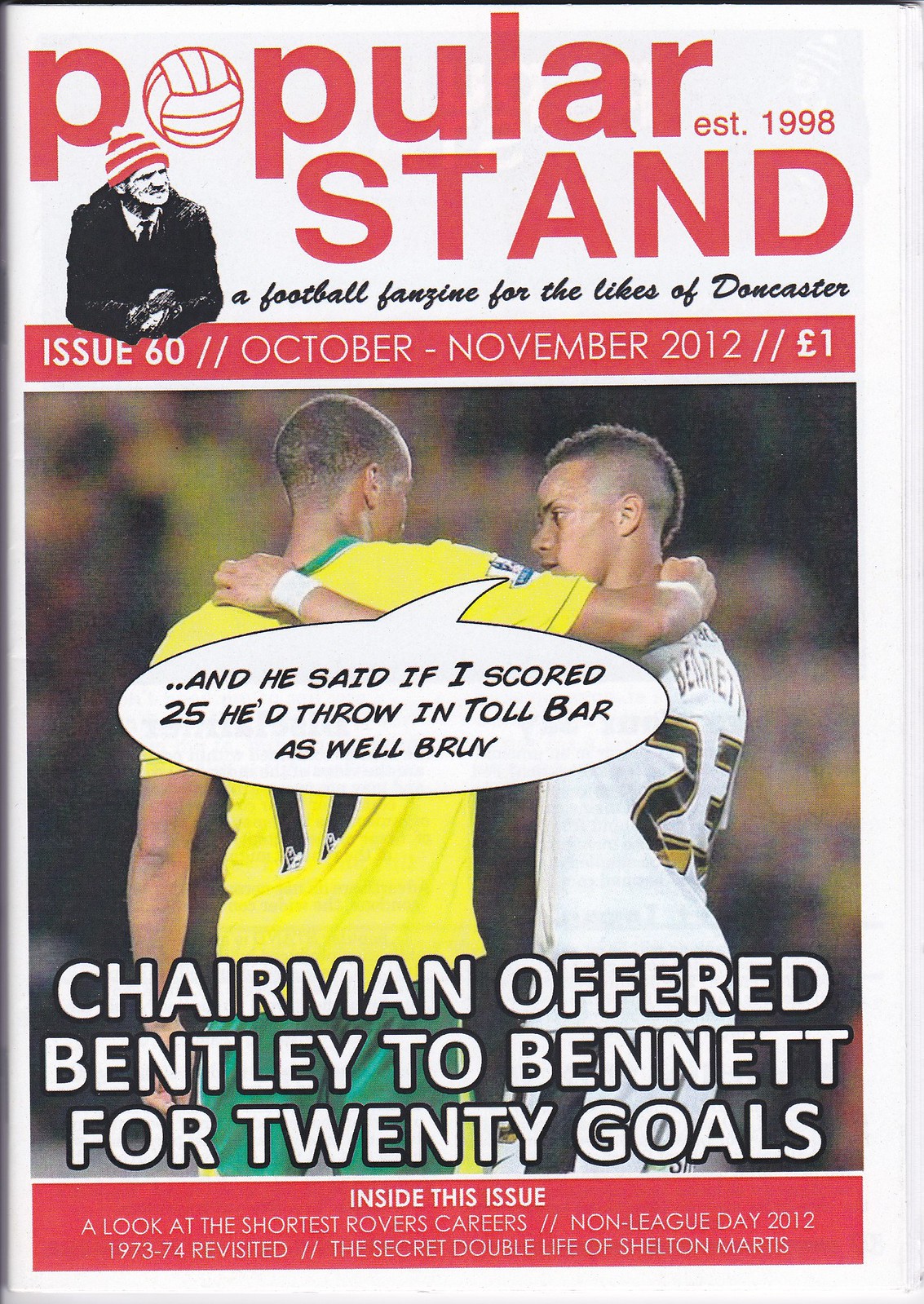The image depicts the front cover of a sports events magazine titled "Popular Stand, EST 1998," designed with a solid white border. The title is prominently displayed at the top in big red letters, with the letter 'O' cleverly replaced by a white soccer ball. Below the title, in smaller black cursive text, it states "a football fanzine for the likes of Doncaster." There's an image of a man wearing a red and white striped beanie with a white poof ball on top, dressed in a black jacket, white shirt, and black tie. Further down, within a red bar, the issue details are mentioned in white font: "Issue 60, October-November 2012," priced at 1 pound. The center of the cover features an illustration of two football players with their arms around each other, accompanied by a thought bubble that reads, "And he said if I scored 25, he'd throw in Toll Bar as well, bruv." Beneath this, it says, "Chairman offered Bentley to Bennett for 20 goals." At the very bottom, another red bar lists the issue's content in white text: "Inside this issue: a look at the shortest Rovers careers, non-league day 2012, 1973 to 74 revisited, the secret double life of Shelton Murtis." The overall design combines various colors, including red, white, green, yellow, brown, black, and gray, giving it a vibrant and eclectic appearance.